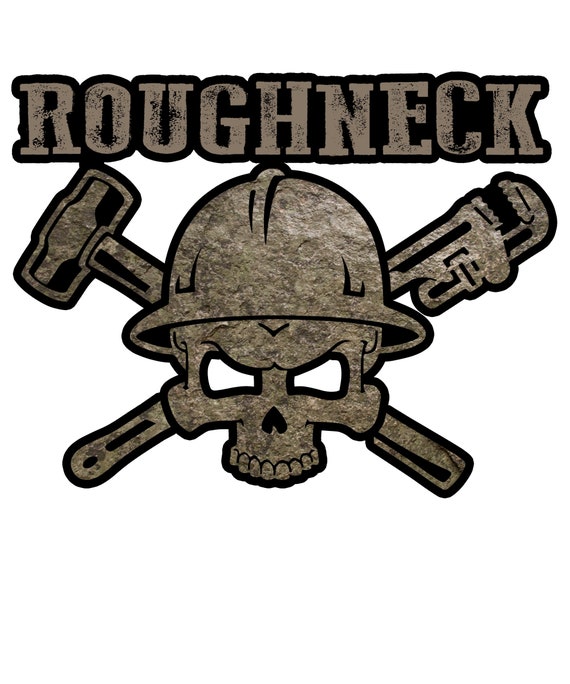This detailed close-up image displays a rugged logo featuring the word “ROUGHNECK” at the top in brown, capital letters with a weathered, rustic appearance, and a shadowed, black outline. Beneath the word, a highly textured, rock-like skull takes center stage. The skull’s fierce expression is highlighted by an angulated V-shaped brow above two exaggerated, downward-sloping brows, and eyeless sockets formed by truncated trapezoids. Its nose resembles an upside-down heart, with an outlined row of teeth but no visible lower jaw. Flanking the skull’s cheeks are two cylindrical protrusions. Adding to its gritty persona, the skull dons a hard hat accentuated with ridges on the top and sides. Emerging from the hard hat are two tools crossing behind the skull: a mallet-shaped hammer on the left and a crescent wrench on the right. The overall image embraces a monochromatic brown hue, accentuating its tough, industrial theme.